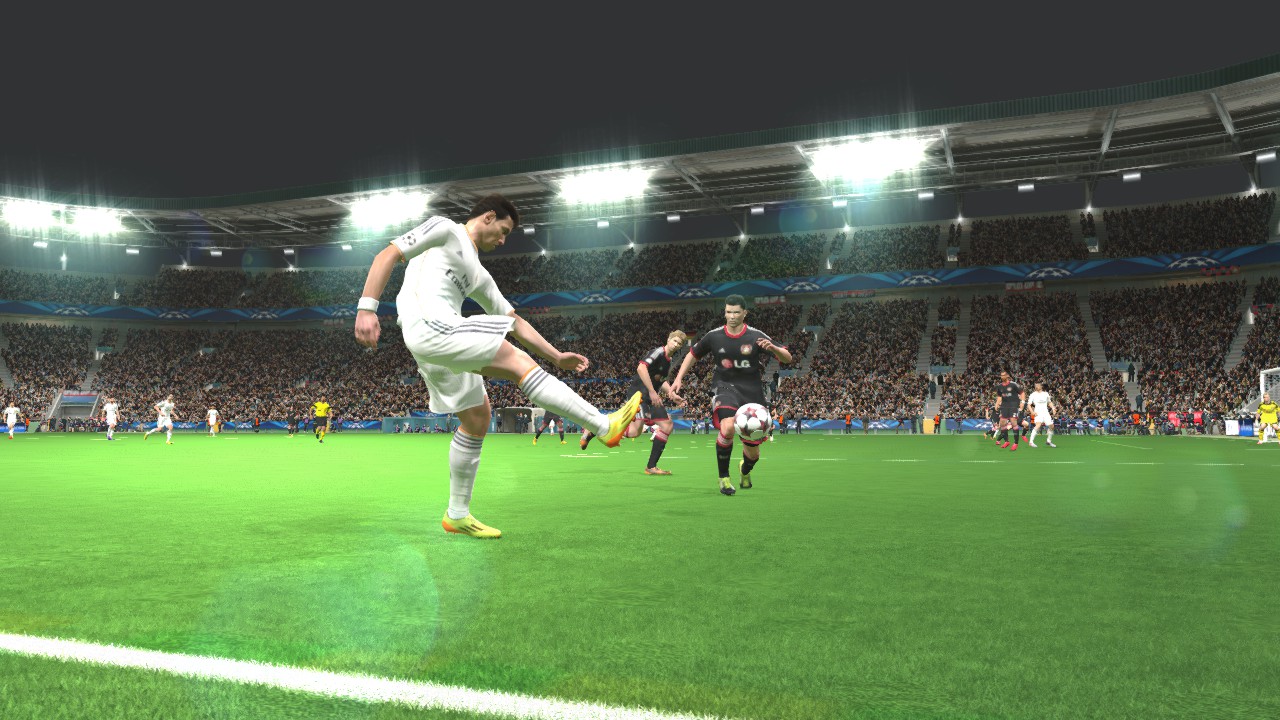The image depicts a dynamic scene from a European football (soccer) match, resembling a detailed video game rendering. Central to the frame is a white soccer ball adorned with black stars. A player dressed in a white outfit with gray vertical stripes on the shorts, white socks, and striking yellow shoes stands poised on the lush green turf. Approaching him is another player clad in black shorts marked with a red line and a black jersey featuring the LG logo in white letters, accented with red trim.

The player in black is intently moving towards the ball which the player in white appears ready to kick. A white line on the turf is visible near the player in white, adding to the field's realism. In the background, there are additional players wearing various outfits in white, black, and yellow. The scene is set within a stadium filled with an animated crowd. Above the stands, stadium lights mounted on a pavilion illuminate the field, enhancing the lifelike atmosphere of the game.